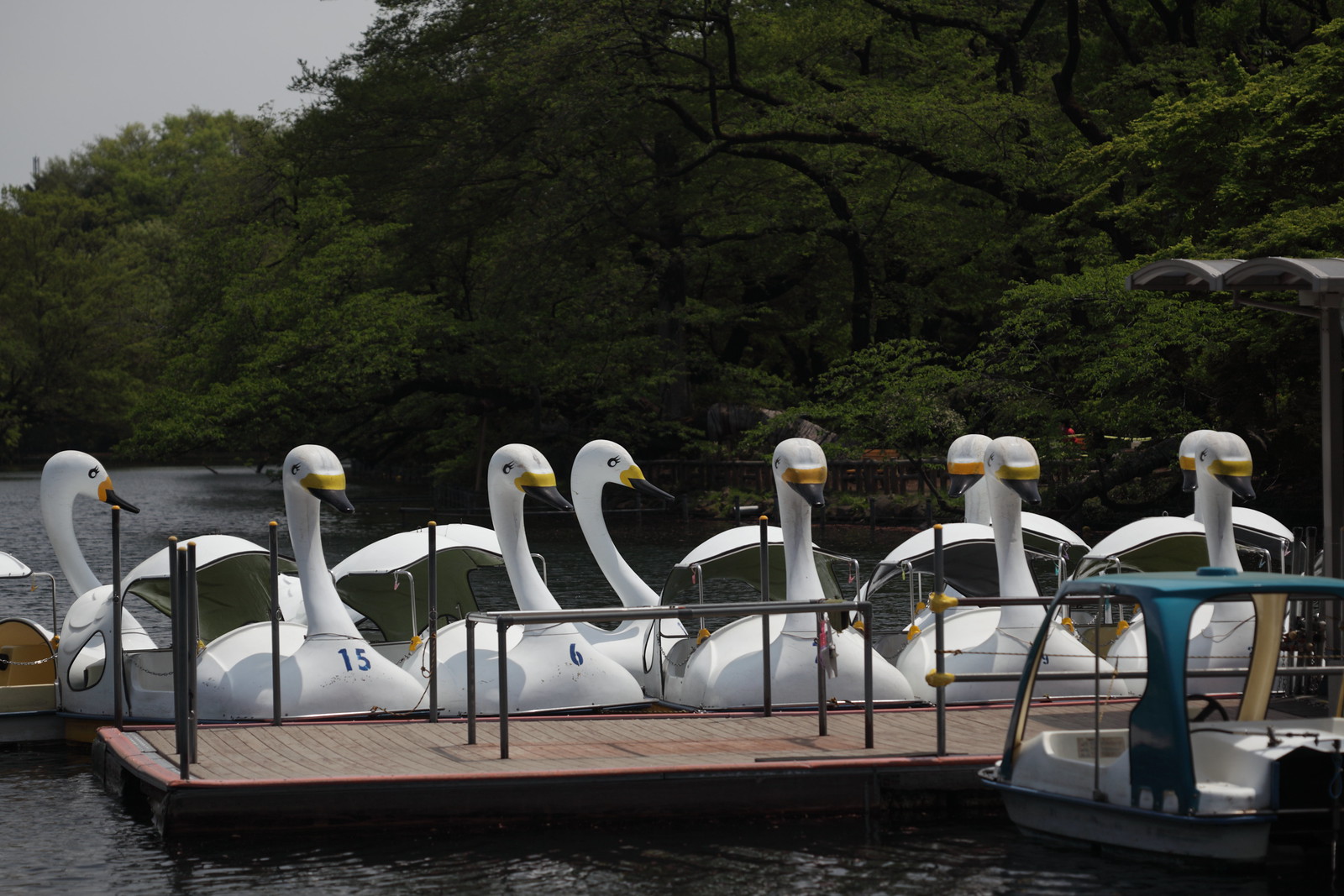In this outdoor photograph taken at a lake, the focal point is a long wooden dock with black and yellow safety railings. The overcast sky, a muted slate gray, contrasts with the dark green trees and bushes that line the lake's perimeter. The dock stretches into the water, where multiple paddleboats are moored. On the right side of the dock, a small white paddleboat with a turquoise-blue roof is visible. Dominating the scene on the left side of the dock are approximately a dozen swan-shaped paddleboats. These white boats feature long necks, black eyes, yellow and black beaks, and roofed seating areas. Each swan boat is individually numbered, with numbers like 6 and 15 clearly visible. The overall atmosphere is serene yet slightly muted by the overcast conditions.